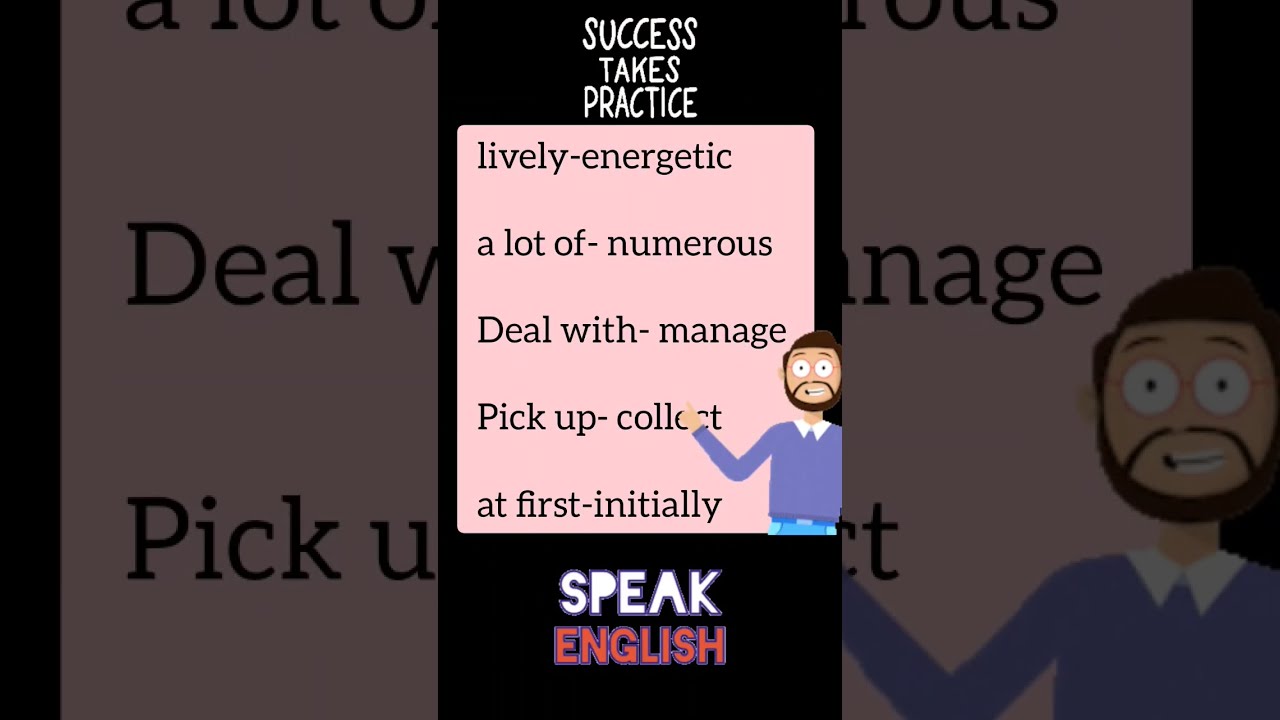The image is an educational cartoon divided into three parts, with the main picture in the center flanked by zoomed-in views of its left and right edges. In the center, there's a rectangular image with a black background at the top and bottom. The top section has three lines of white text that read, "Success takes practice." Below this, there's a prominent pink box containing the words "lively, energetic, a lot of, numerous, deal with, manage, pick up, collect, at first, initially" in black font. 

A cartoon character, positioned on the right side of the pink box, appears to be engaging with the text. He sports a blue sweater over a white-collared shirt, has brown hair, a brown beard, and mustache, with large white-rimmed glasses and tiny pupils. His arm is extended, pointing towards the section that says "pick up, collect." 

At the bottom of the pink box, there's another section in white text with a bluish border that reads "speak English," followed by additional text in red with a blue border. The zoomed-in views on the left and right edges highlight different parts of the central image, further capturing sections of the text and parts of the cartoon character’s upper body.